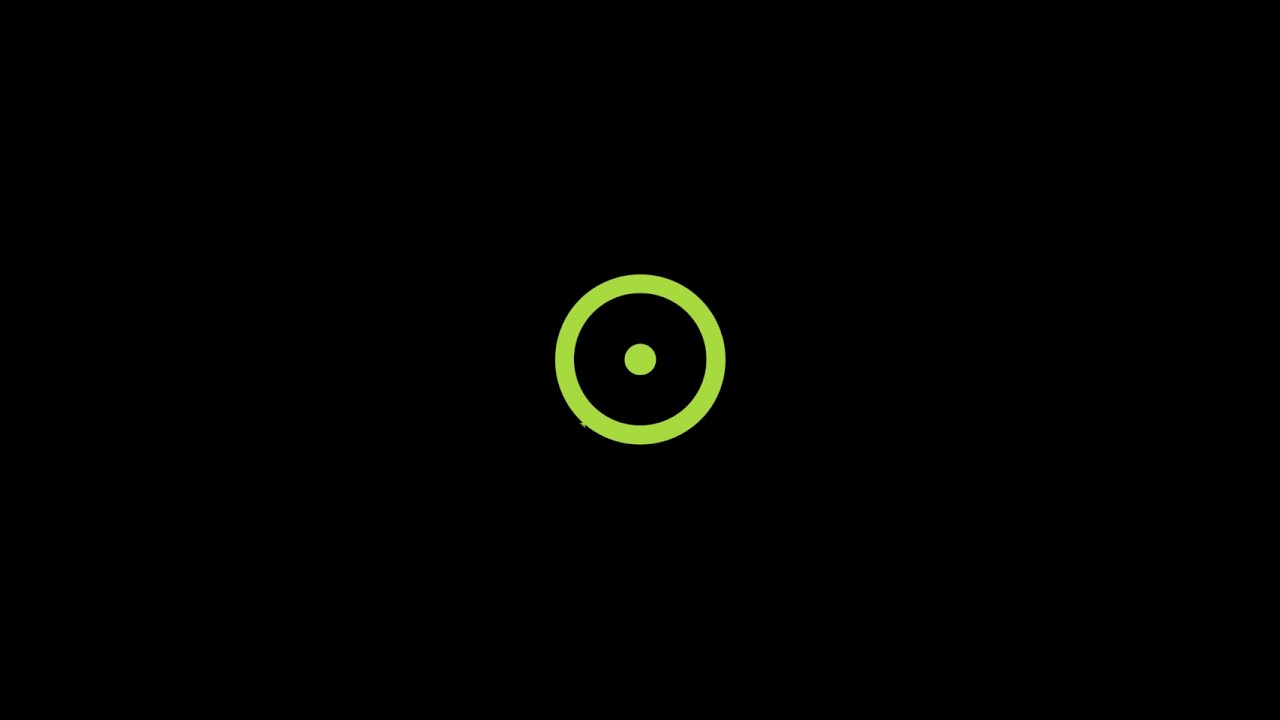The image features a simple, centrally positioned logo set against a pitch-black background. The logo itself consists of a light green dot at its core, encircled by a larger light green ring, similar to a target or a donut shape with a black space between the central dot and the outer ring. Upon close inspection, there is a discernible small protrusion on the otherwise perfectly circular outer ring, suggesting a minor design flaw. The entire composition is devoid of any additional text or imagery, emphasizing the stark contrast between the light green and black hues.